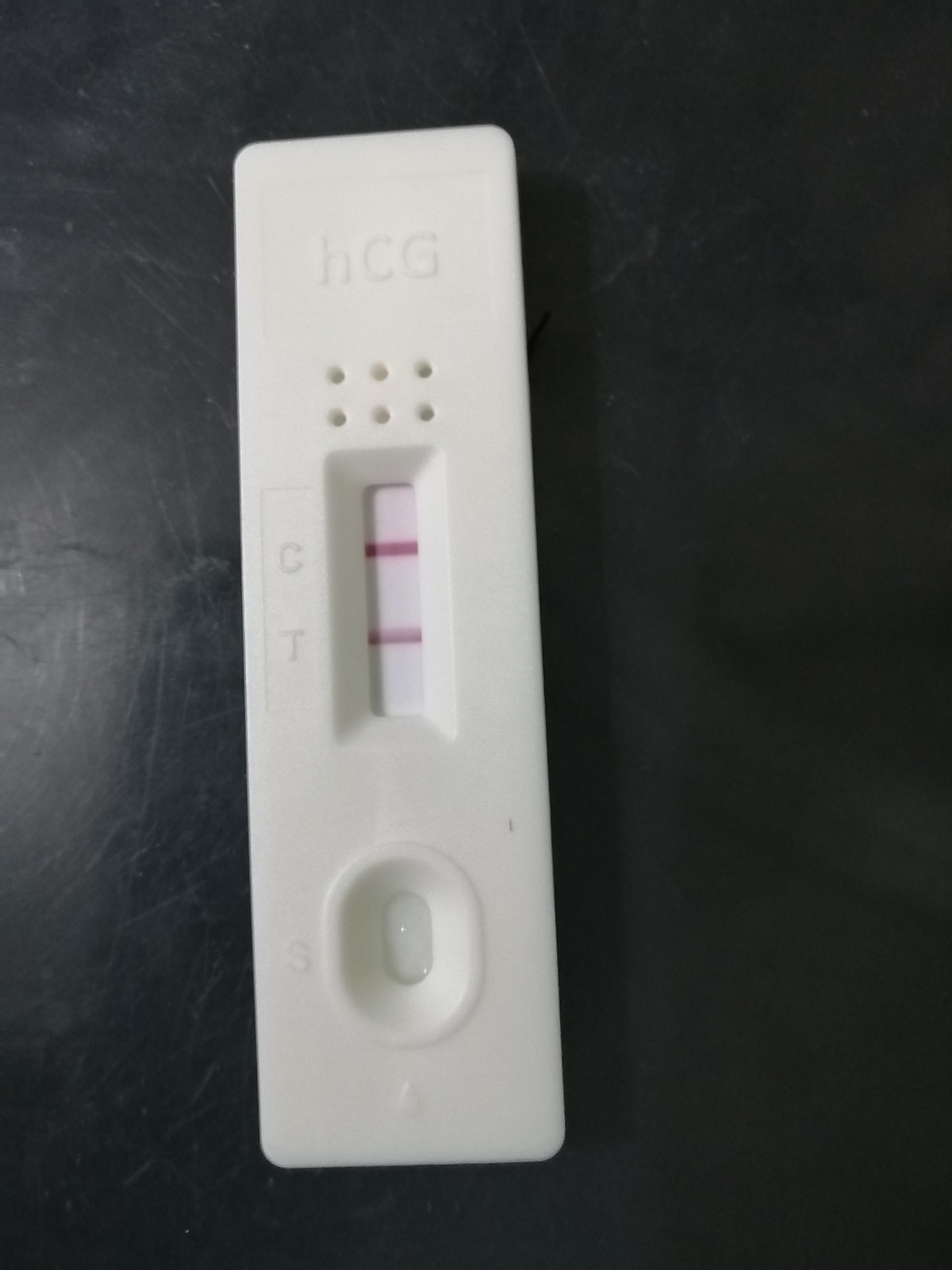This image features a white rectangular test strip placed on a textured, matte black surface, which appears to be the cushion of a chair or stool, likely made of leather or vinyl. The test strip has a matte white finish and displays a series of markings. At the very top, there are three letters: a lowercase "h," followed by uppercase "C" and "G." Below these letters, there are two rows of small circular holes, resembling the size of a toothpick puncture – three holes in each row, totaling six.

In the center of the test strip, there is a small screen displaying two pink lines. The top line is solid, labeled with a "C" to its left, and the lower line is faded, labeled with a "T." At the bottom of the strip, there is a round-shaped area with a small white hole, marked with an "S" to its left and a droplet symbol beneath it, indicating where a sample is to be placed.